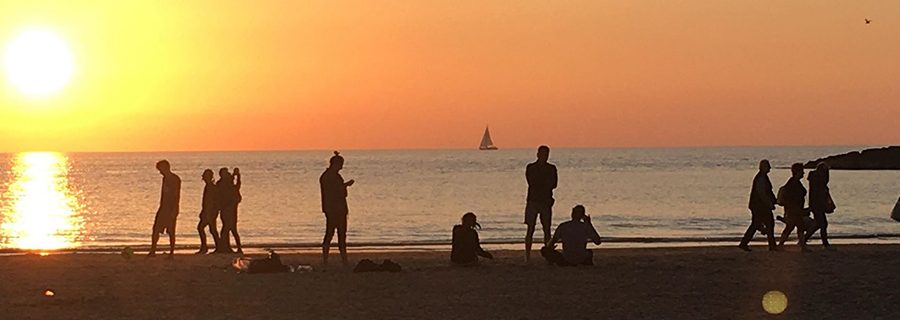A wide, panoramic, color photograph captures a serene beach scene at sunset with an array of silhouetted figures. On the far left, the sun, large and glowing orange, is near the horizon, casting a long, reflective trail of light across the calm ocean waters. In the foreground, the golden sand is dotted with approximately ten people: some walking in both directions, others sitting or standing, and a few capturing the picturesque moment on their phones. A man is seen playing with a soccer ball while another appears to be engrossed in his phone. At the center of the image, distant on the horizon, sails a solitary boat. Towards the right of the frame, a group of three individuals are carrying folding beach chairs, departing the sunset scene. Also visible on the right is a rock jetty jutting out into the water and, overhead, a lone bird is flying. The sky is awash with hues of orange, seamlessly blending into the calm blue of the sea, creating a tranquil and evocative atmosphere. The low sun’s light has also caused a slight lens flare at the bottom right of the image, adding to the photograph’s serene yet dynamic charm.